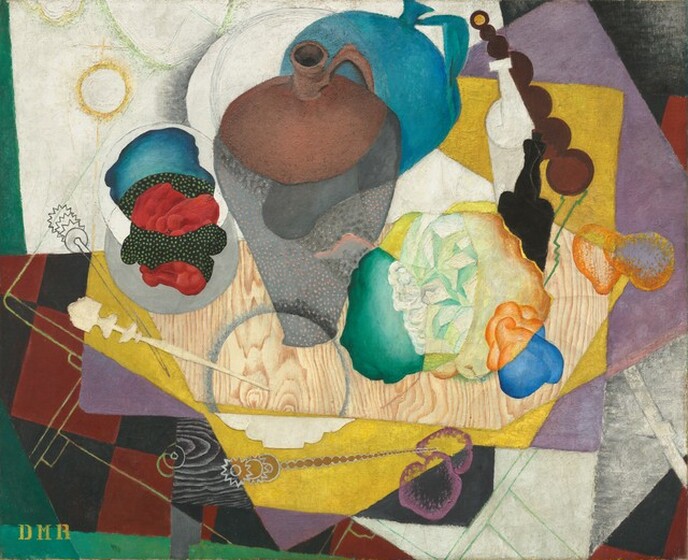The image is a highly detailed, colorful painting exhibiting a collage-like composition with multiple layered elements and abstract shapes. Dominating the composition is a central vase or urn, characterized by a clear gray body, a brown top, and a jug-like handle, alongside another canteen-like object in blue. The background is a multi-layered tapestry of colors including dark green, dark gray, red, purple, burgundy, yellow, orange, teal, blue, and white. Notable patterns include marble-like textures, blocks of purple and blue, yellow squares, a red and black checkered design, as well as segments resembling wood grain. Toward the bottom, the painting features white paper with lines and yellow-orange paper with purple tips. More abstract, circular shapes and wooden textures are dispersed throughout. The painting is signed with the initials "DMR" in yellow located in the lower left-hand corner, indicative of the artist's mark.